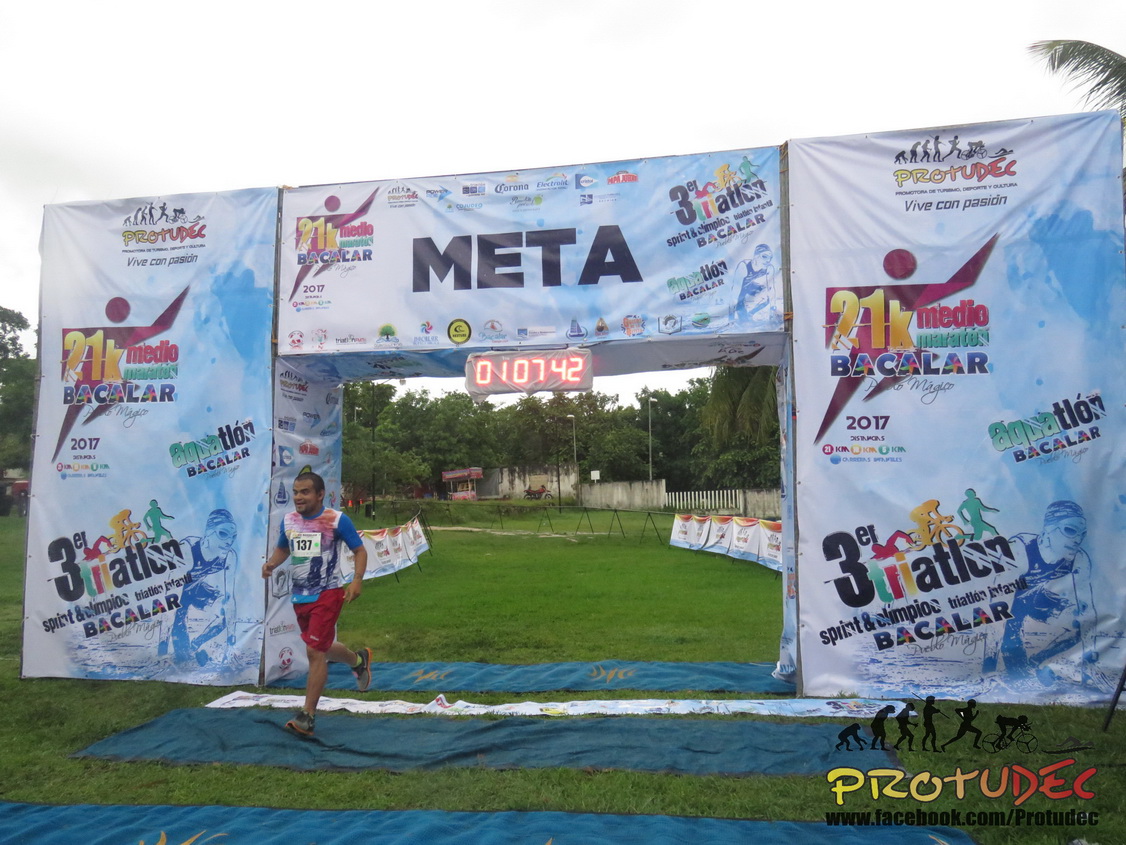In the image, a runner is crossing the finish line of a marathon, specifically a 21K Medio Marathon Bacalar, amidst a scenic, green setting. The finish line features a square archway adorned with promotional banners on a white to light blue background, bearing various sponsor logos, including Bacalar Media. The top of the arch prominently displays the word "META" in dark blue text. A digital clock, hanging from the center of the archway, shows a time of 1:07:42. The runner, wearing a blue, red, and white graphic shirt with red shorts and shoes, is captured mid-stride under the arch. He wears a paper bib number "137" on his chest. The pathway to the finish line is a grass lane bordered by white banners and flanked by barricades. In the lower right corner of the image, there is a logo that spells "PROTUDEC". The background reveals a forest with numerous trees under an overcast sky, and a white fence bordering the forest area. No other runners are visible in the picture.